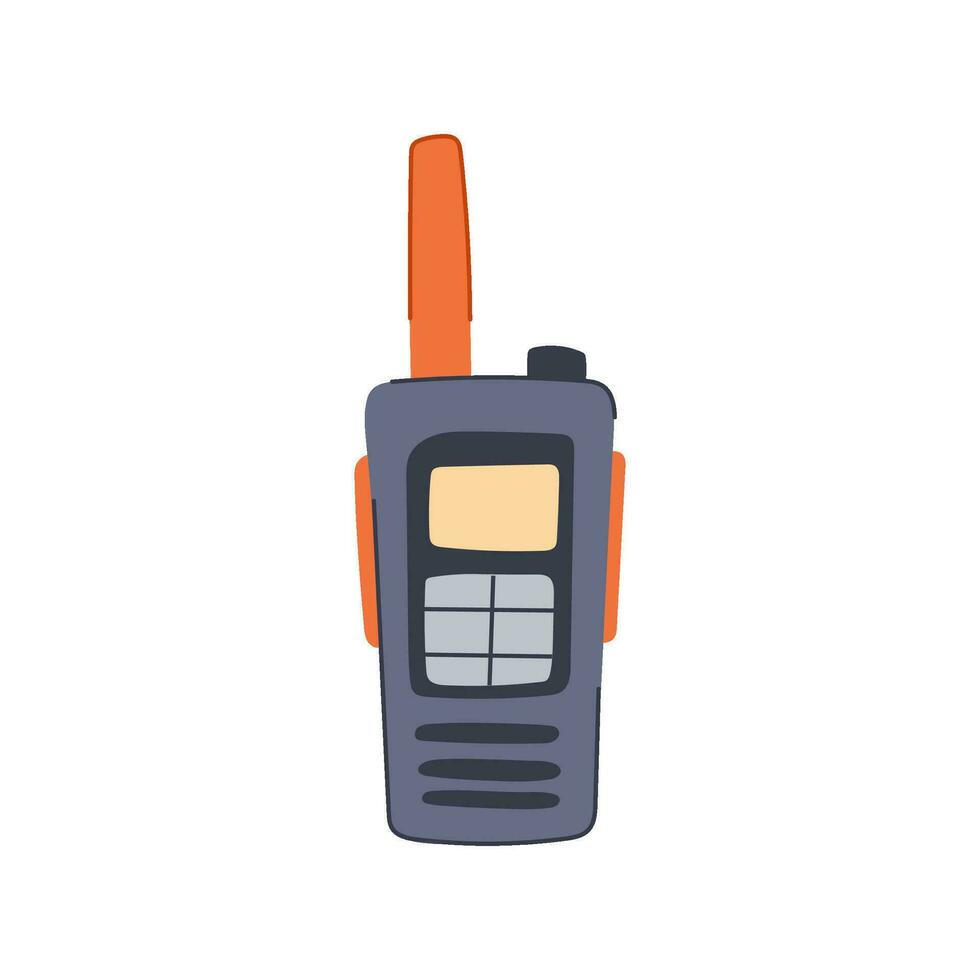This image depicts a digital graphic of a walkie-talkie on a white background. The walkie-talkie has a vertically oriented, rectangular body with a bluish-gray color. In the center of the rectangle, there is a smaller vertical dark gray rectangle. This contains a horizontally oriented yellow screen. Below the screen, there is a white square divided into six sections, likely resembling some form of buttons or a keypad. Further down, three vertical dark gray lines represent audio lines or a speaker. Prominent orange accents are present, with two orange lines on each side of the body forming buttons, and a thick orange antenna protruding from the top left side. Adjacent to the antenna on the top right, there's a small circular black knob. The design is simple yet detailed, making the walkie-talkie the focal point of the image without any background distractions.